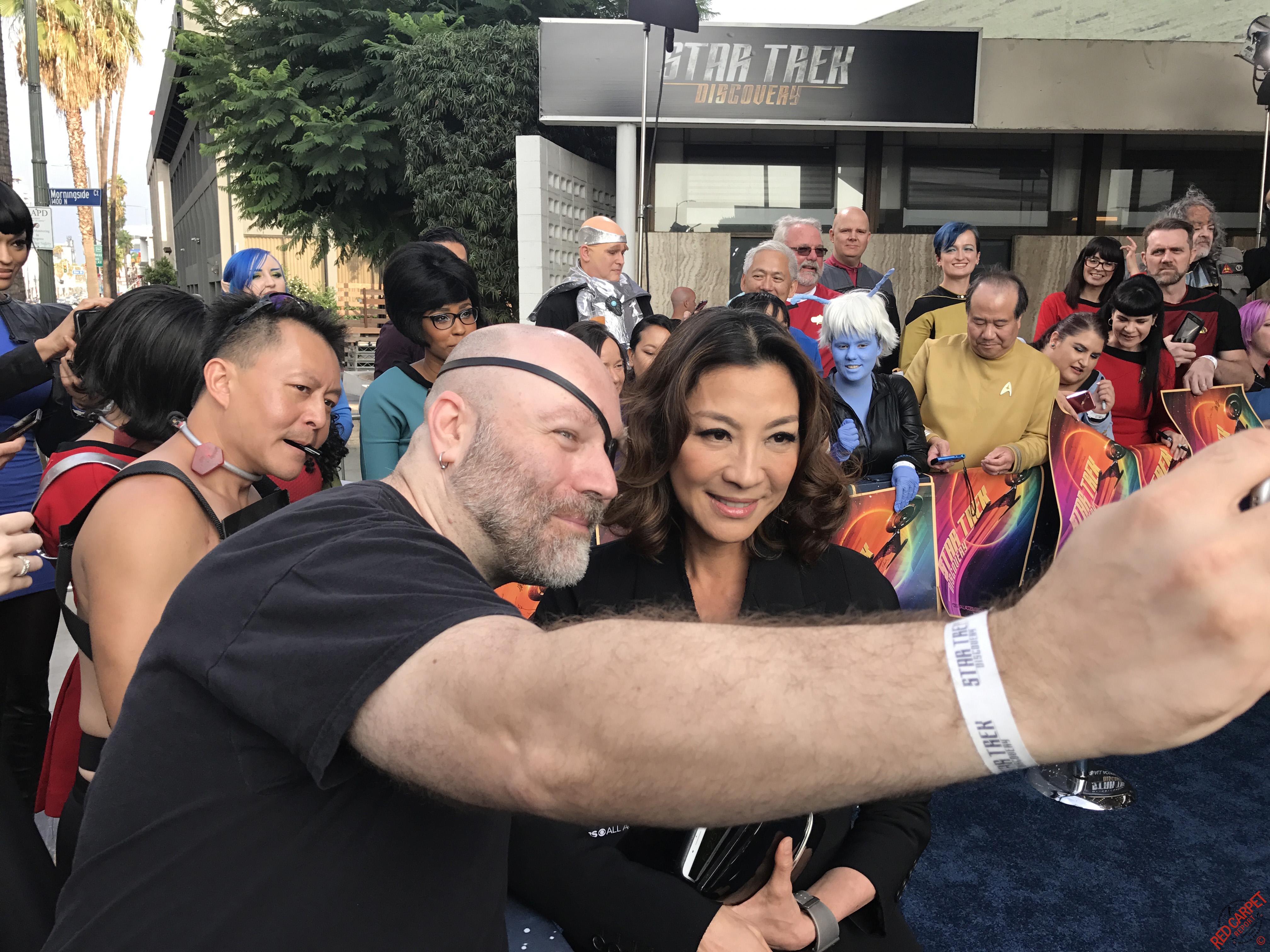At what appears to be a premiere event for a Star Trek sequel, a man stands on a blue carpet in the center of the image, extending his arm to take a selfie. He wears a black shirt and has a distinctive black eyepatch over his left eye. His right hand is adorned with a white ribbon, potentially related to the Star Trek theme. Flanking him on either side are two individuals: to his left, an Asian woman in her 50s with a medium-curled hairstyle, dressed in a black suit and sporting a watch on her left wrist; to his right, an Asian man in his late 40s or early 50s, donning a black tank top and wearing an unidentified item around his neck. In the background, a large Star Trek banner hangs on a building, hinting at the nature of the event. A crowd dressed in Star Wars costumes stands behind a barricade, adding to the festive and sci-fi themed atmosphere.